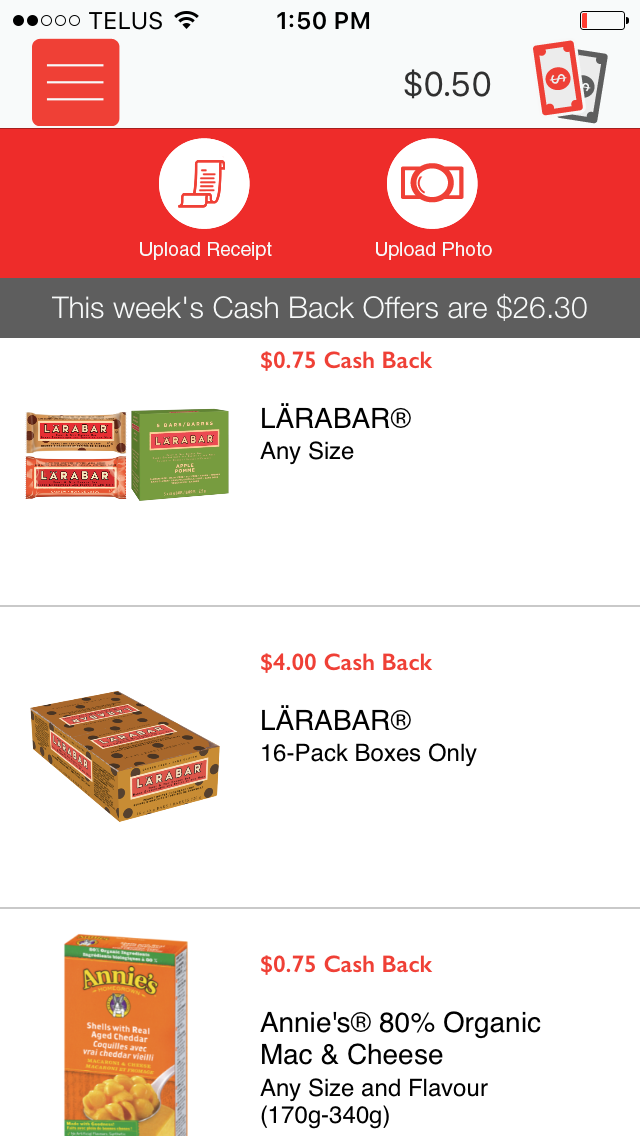This is a detailed screenshot from a shopping website, likely displaying cash back offers. The top of the image features the word "TELUS" along with a Wi-Fi symbol, two black circles, and the time displayed as 1:50 PM. Additionally, a battery icon is visible.

Below this, there is a red box with three white lines and text in black displaying "$0.50". Adjacent to this text is a red and black dollar bill icon.

Further down, a red box includes two red and white circular buttons. The first button says "Upload Receipt" and features a receipt icon, while the second says "Upload Photo" with a camera icon.

Continuing down, gray and white text announces, "This week's cash back offers are $26.30".

The main section includes three white boxes, each presenting a different product with corresponding cash back offers. The first box advertises "$0.75 cash back" on any size of Larabar, accompanied by an image of green-packaged Larabars. The second box offers "$4 cash back" for Larabar 16-pack boxes, shown in a gold package filled with bars. The third box promotes "$0.75 cash back" on Annie's 80% organic mac and cheese, applicable for any size and flavor ranging from 170g to 340g, with an image of the product.

Characteristics such as gray bars between product descriptions, bold and easy-to-read fonts, and a clear, user-friendly interface complete the image.